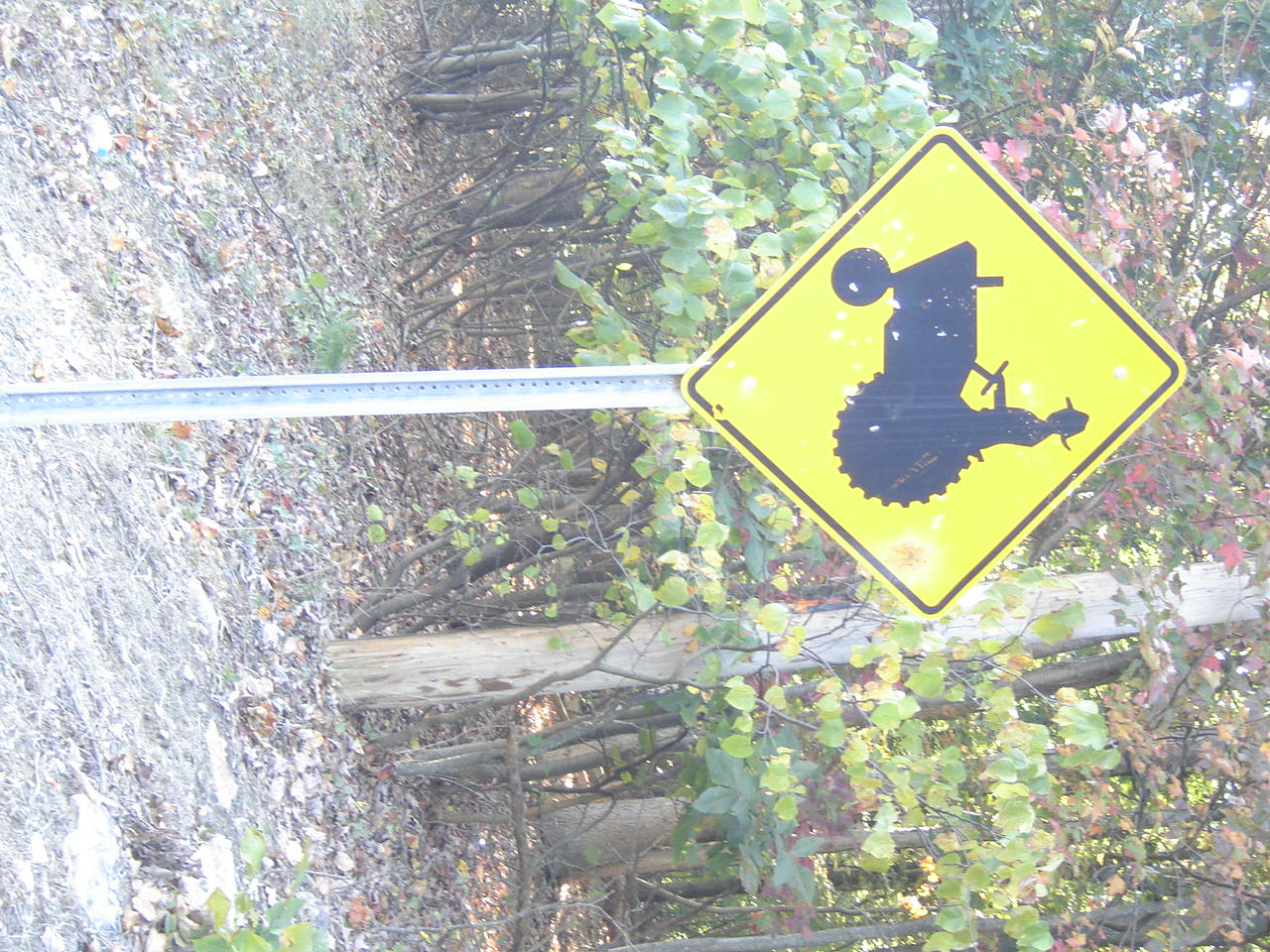This outdoor photograph, which has been rotated sideways with the top now on the right-hand side, depicts a richly detailed scene. The right side of the image features a tree line where the foliage transitions from reddish hues at the top to green shades below, with the brown trunks at the base. The left side showcases a dirt ground interspersed with dead leaves, patches of grass, and hay-like sections. Prominently visible on the left is a silver metal pole bearing a yellow diamond-shaped sign with a silhouette of a person driving a tractor in black. Among the trees in the background, various colored leaves—gray, brown, red, and green—fill the upper portion of the scene, creating a vibrant and textured tableau that suggests careful, purposeful planting.